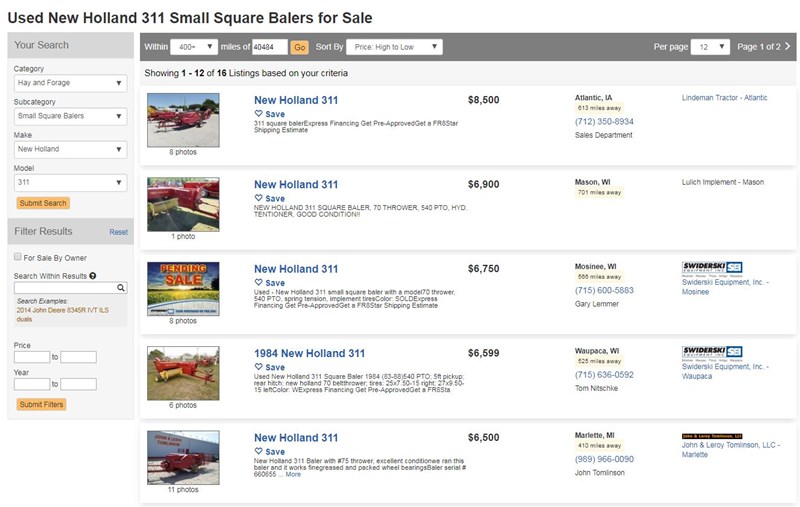The image displays a web page featuring a sales listing for used New Holland 311 small square balers available within a 400-mile radius of postal code 40484. The results are sorted from highest to lowest price and appear on page 1 of 2. 

The listings include:

1. New Holland 311 priced at $8,500, featuring "Save 311" and options for Express Financing and FRS Star Shipping Estimates.
2. Another New Holland 311 listed for $6,900.
3. A New Holland 311 priced at $6,750.
4. A 1984 New Holland 311 offered for $6,599.
5. Another New Holland 311 available for $6,500.

Each result includes respective phone numbers for further inquiries. On the left side of the page, there are various filters available to refine the search results.